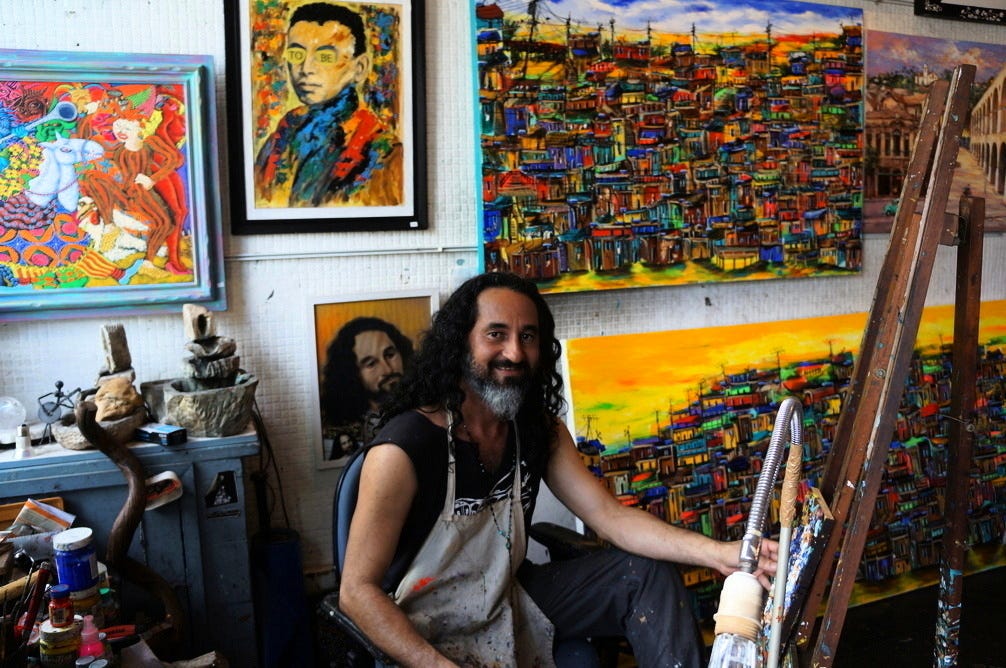The landscape-oriented color photograph captures the vibrant interior of an artist's studio. Dominating the center, near the bottom of the image, is a smiling man seated in a folding chair. He is an artist named Domingos Cardoza, recognized for his work in photographic representationalism realism and hailing from Rio de Janeiro's favelas. Domingos has long, curly black hair and a gray beard, and he wears a beige apron splattered with paint over a black tank top and gray pants. His bare, muscular arms are indicative of someone who frequently engages in manual, creative labor. With a dark-eyed gaze and a welcoming smile, he looks directly at the viewer while his left hand rests on an artist's easel in front of him. Although the small canvas on the easel is out of view, his focus on it is apparent.

Behind him, the backdrop features a white tiled wall adorned with a plethora of colorful pictures and paintings. The artworks exhibit a spectrum of colors, reminiscent of a rainbow, and include a large rectangular wooden table laden with various art supplies. Notably, there are distinctively vivid pieces: one featuring a yellow sky and a sea of multicolored buildings stacked atop each other to the right of Domingos, and another in the middle portraying a man with characteristics strikingly similar to Domingos, suggesting it might be a self-portrait of a younger version of himself. Additional paintings include a lively depiction of a city in the top right and an orange and blue jester in the top left corner, contributing to the chaotic yet vibrant aesthetic of the studio environment.